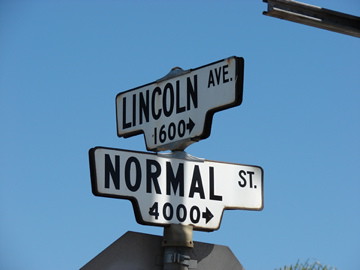The image showcases two white street signs on top of a partially visible silver metal post under a clear blue sky. The focal point is the two signs: the top one reads "Lincoln Avenue, 1600" with an arrow pointing to the right, and the bottom one reads "Normal Street, 4000" (abbreviated as ST.) also with an arrow pointing to the right. Both signs have a distinctive design with a flat top and a slightly angled downward extension at the bottom. Below them, the back edge of what appears to be a stop sign is visible, characterized by its dark gray backside. A black metal beam intrudes from the upper right corner, possibly connected to another sign.